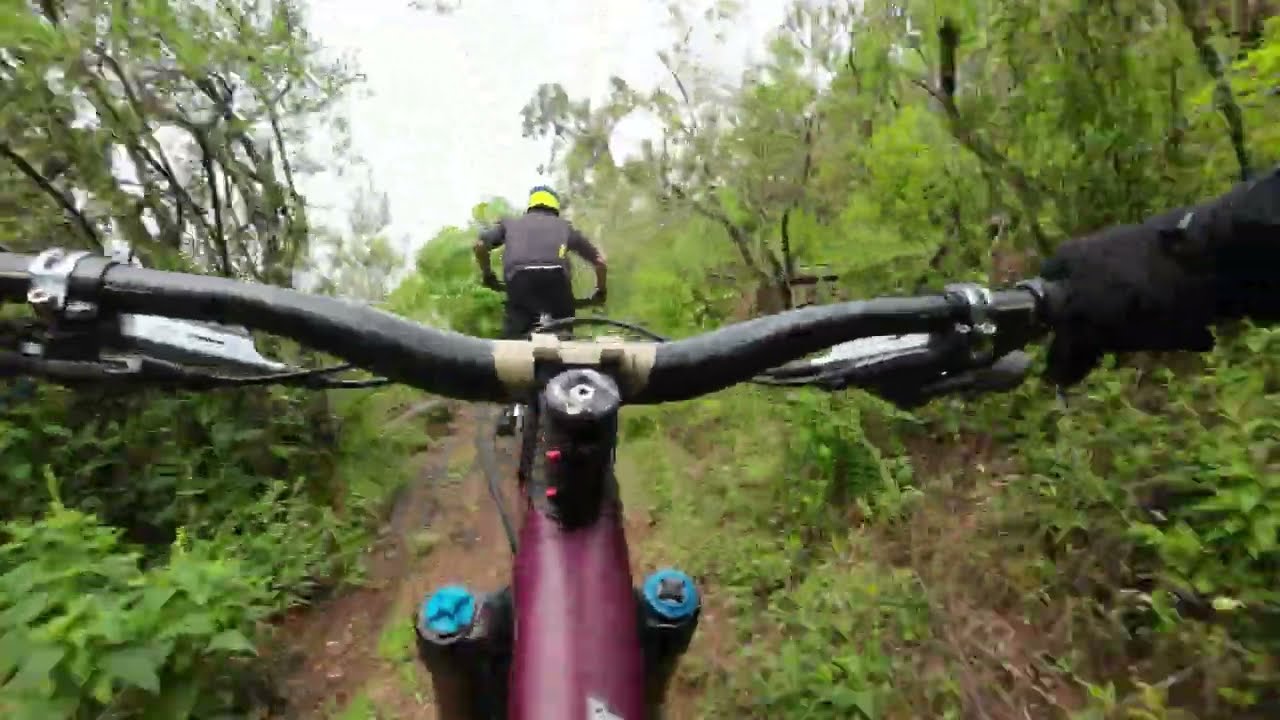This image captures a vibrant and dynamic moment on a mountain biking trail within a lush, green forest. Taken from the vantage point of a bike rider using a GoPro or similar device mounted around the chest area, the image prominently features the maroon frame of the bike with distinct blue bolts near the black handlebars. A gloved hand grips the right handlebar, guiding the bike along a narrow, muddy dirt path which cuts through a verdant landscape dotted with green grass, small trees, and ferns. 

Leading the way on the trail is another cyclist, identifiable by their yellow helmet, gray sweatshirt, and black pants, who is seen navigating the twisting path ahead. A bright, overcast sky casts a diffuse white light over the scene, illuminating the lush surroundings and adding a natural glow to the terrain. The pathway, winding sharply to the right at the top of the image, underscores the adventurous and invigorating essence of this forest ride.